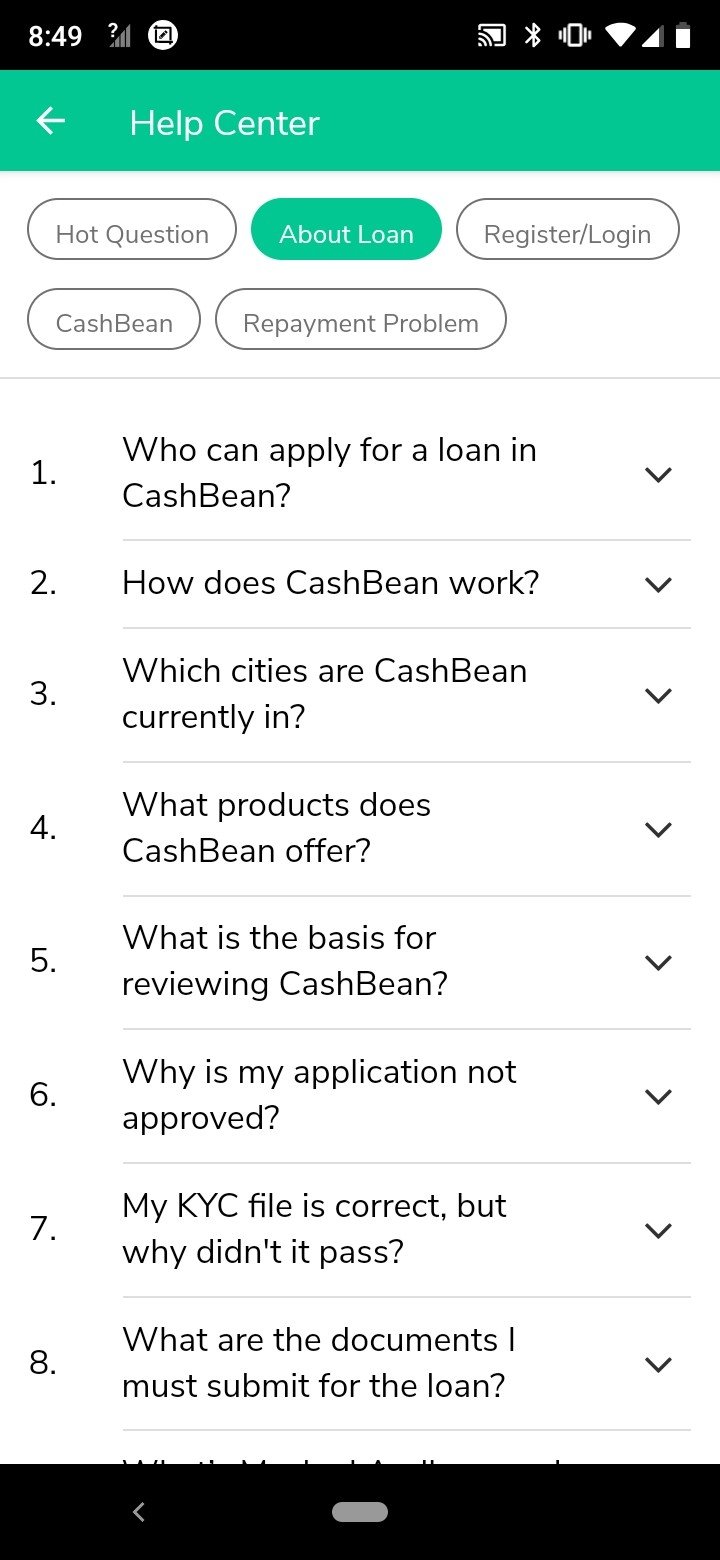This screenshot from a smartphone captures a detailed view within the Cash Bean app's Help Center. At the very top of the image, a black toolbar displays the current time, 8:49, with indicators showing full bars of cellular signal, a strong Wi-Fi connection, a fully charged battery, and volume turned up. Below this toolbar, a light blue-tealish banner prominently displays the label "Help Center." The user is currently in the "About Loan" section of the Help Center, which offers eight different informational areas. These sections include queries like "Who can apply for a loan in Cash Bean?" and "How does Cash Bean work?" The bottom of the screen features another black toolbar with a left-pointing arrow for navigation. The overall background of the interface is a clean white color, with all text in black for easy readability.